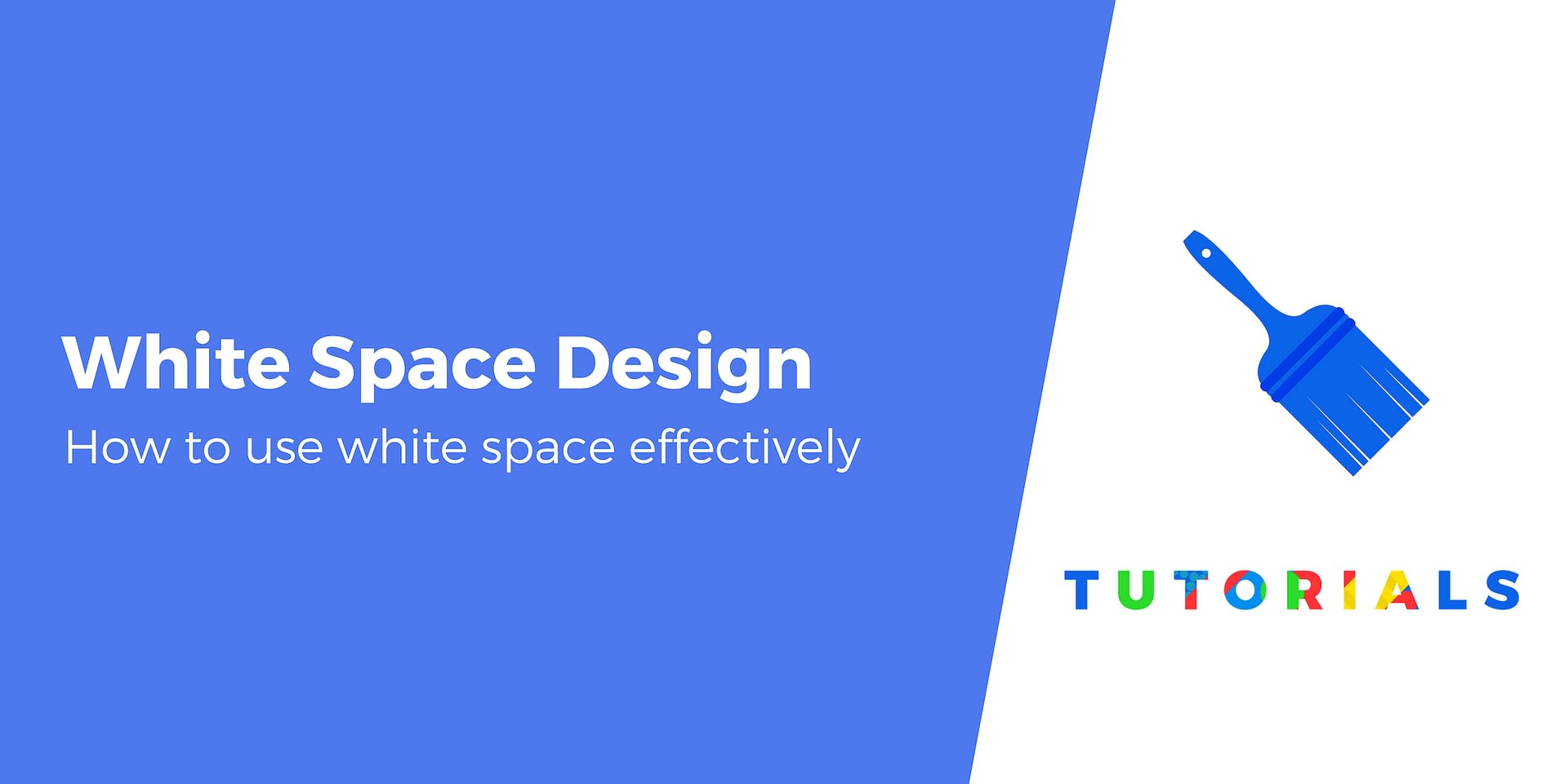The slide presents a detailed tutorial on white space design, structured with a blue-dominated, rectangular layout. The left section, occupying two-thirds of the image, features a vibrant blue background with prominent white text. At the top, a headline reads "White Space Design," followed by a subheading, "How to Use White Space Effectively." On the right side, a diagonal slash separates the segments, transitioning to a white background. This section showcases a blue graphic of a paintbrush pointing diagonally towards the bottom-right corner. Just beneath the graphic, the word "TUTORIALS" stands out in bold, multicolored capital letters, with each letter varying in blue, green, red, and yellow hues, creating a vibrant, scattered effect.